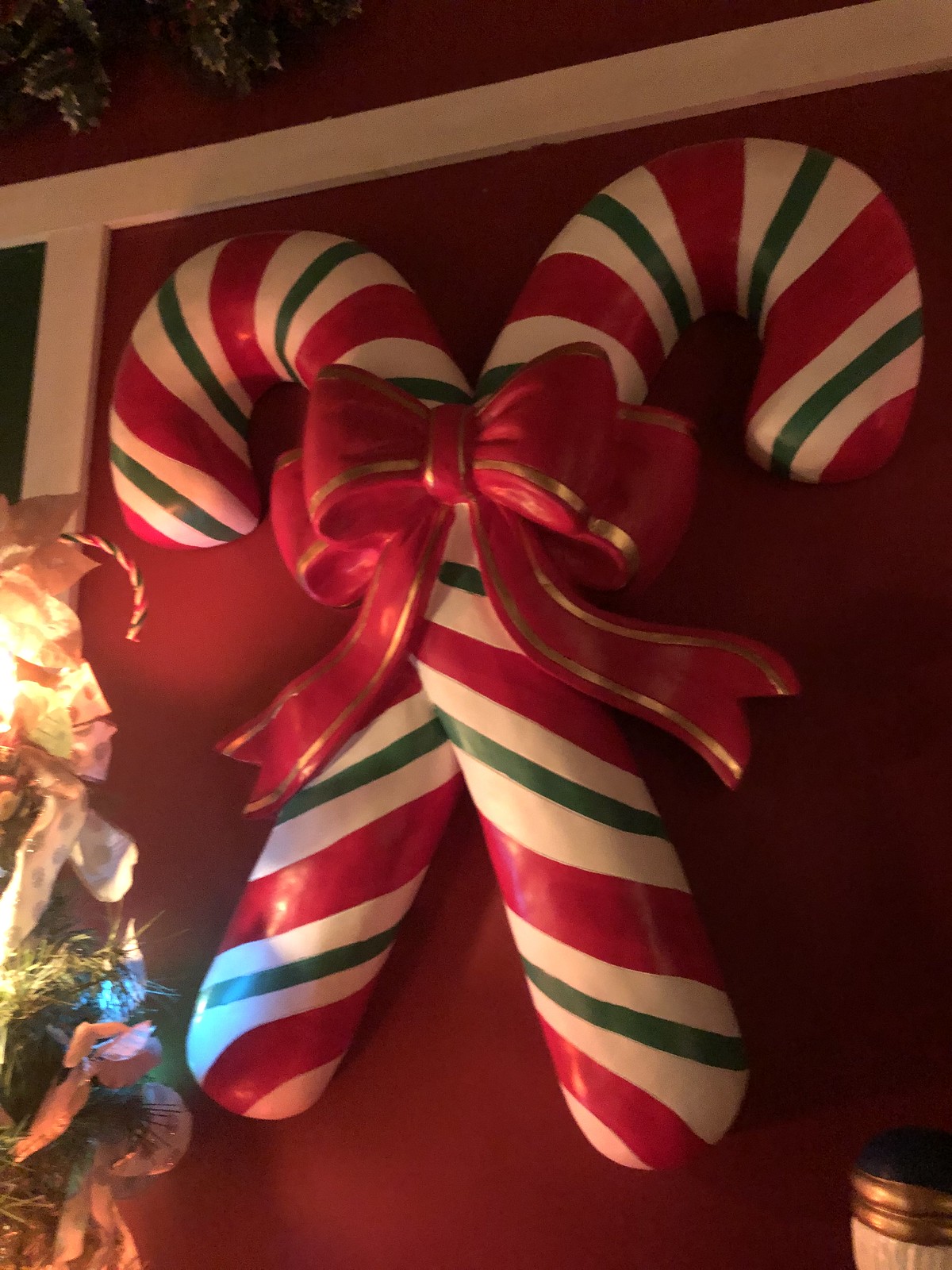This photo shows a striking indoor display of two very large, crisscrossed candy cane decorations mounted against a red wall with white trim. Each candy cane features bold diagonal stripes in white, red, and green, and they are tied together at the center with a generous red and gold bow. The candy canes are angled opposite each other, with their hooks extending to the left and right, creating a balanced visual effect. In the lower left corner, a Christmas tree adorned with lights adds a festive touch, its size highlighting the impressive scale of the candy canes. A partially visible green wreath with lace ribbon can be seen to the right of the display, along with some gold Christmas ornamentation in the lower right corner. There is a soft glow cast on the candy canes, presumably from a nearby lamp, enhancing the cozy holiday atmosphere.